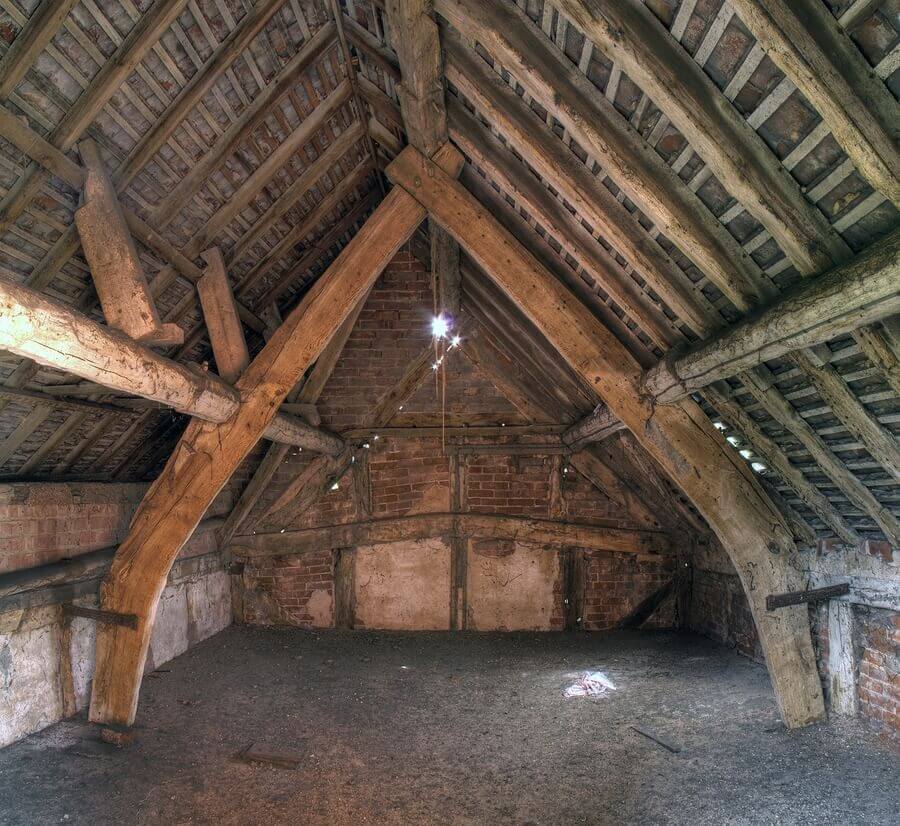The image depicts the interior of an old, weathered attic with a pitched roof. The roof structure is supported by wooden rafters and beams forming an inverted V shape, stabilized by crosswise pieces of wood. The attic has no insulation, allowing a clear view of the wooden framework extending up to the roof. The walls on the left and right, as well as at the far end, are constructed of very old, worn bricks, presenting a reddish, orangish hue. The floor is covered with what appears to be a gray carpet. At the peak of the far wall, there is a light shining into the attic. The overall appearance suggests that the attic is at least from the early 1800s, characterized by faded wood and brickwork, contributing to its antique and rustic ambiance.